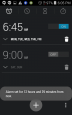This screenshot, captured from a mobile device, exhibits a notably low-quality image, characterized by a pronounced blur that renders finer details indistinct but still recognizable due to the familiar nature of the device. The image has been cropped to focus solely on a specific section of information, yet it retains the typical icons found at the top of a phone screen, including messaging app notifications, the time, battery status, and network connections.

In this particular screenshot, the phone's clock function is displayed, showcasing features such as alarm settings, timers, and stopwatches. The visible alarms detail that an alarm has been set for 6:45 AM, activated for five days of the week. Another alarm is visible, set for 9:00 AM, though it is currently switched off and scheduled exclusively for Saturday and Sunday. At the bottom of the screen, there is a prominent grey circular plus button, providing the option to add new alarms.